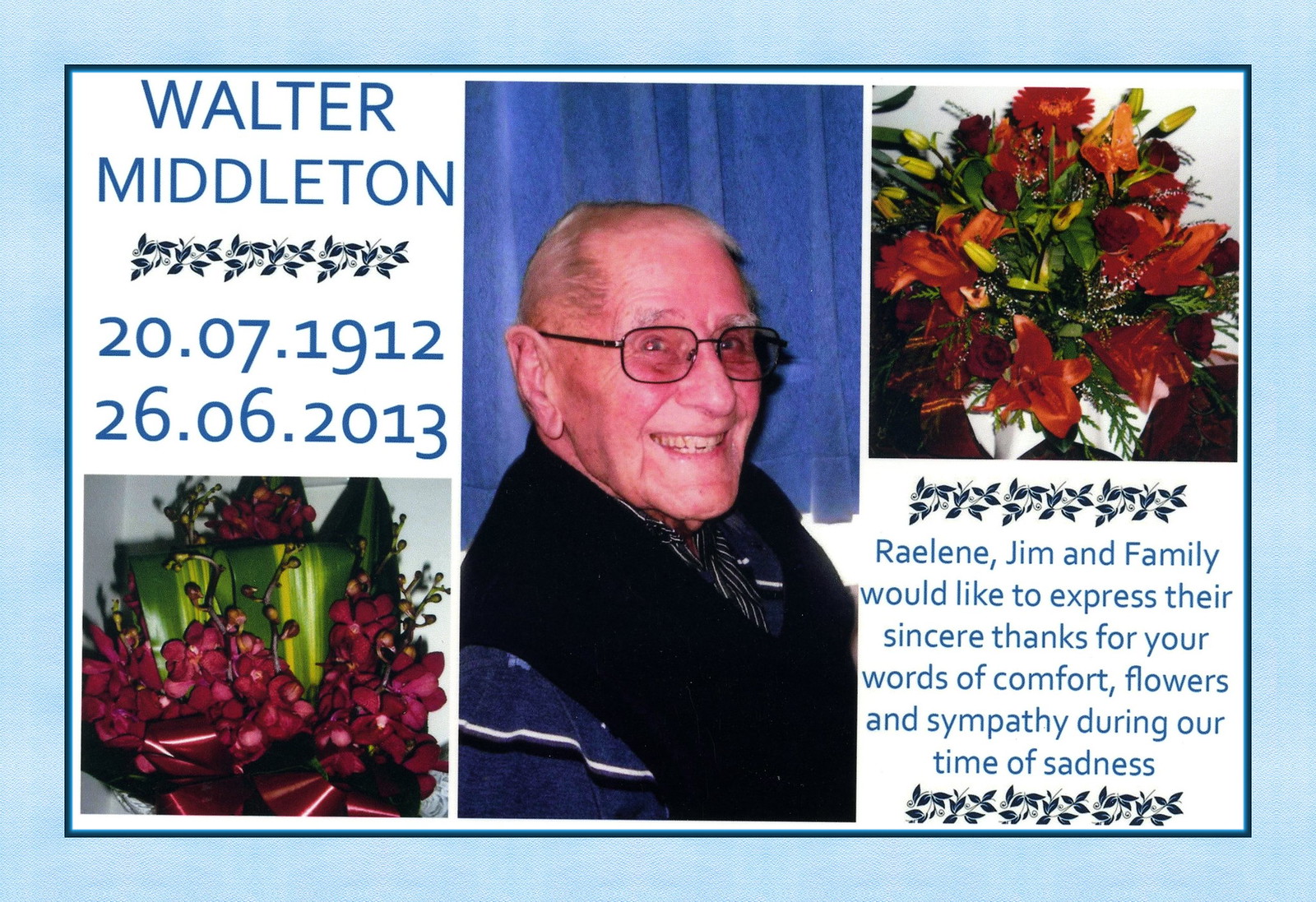This colorful collage serves as an obituary announcement for Walter Middleton. At the center is a touching photo of an elderly gentleman, donned in black glasses, a blue shirt with black and white stripes, and a black sweater vest. He is smiling warmly at the camera. To the right of the photograph is a beautiful bouquet of flowers, while another arrangement adorned with a red ribbon is seen below the dates on the left. The large text on the left reads "Walter Middleton, 1912-2007, 26-06-2013," marking his birth and passing dates. The sincere message on the right from Raylene, Jim, and their family extends heartfelt gratitude for the comforting words, flowers, and sympathy received during their time of sadness.